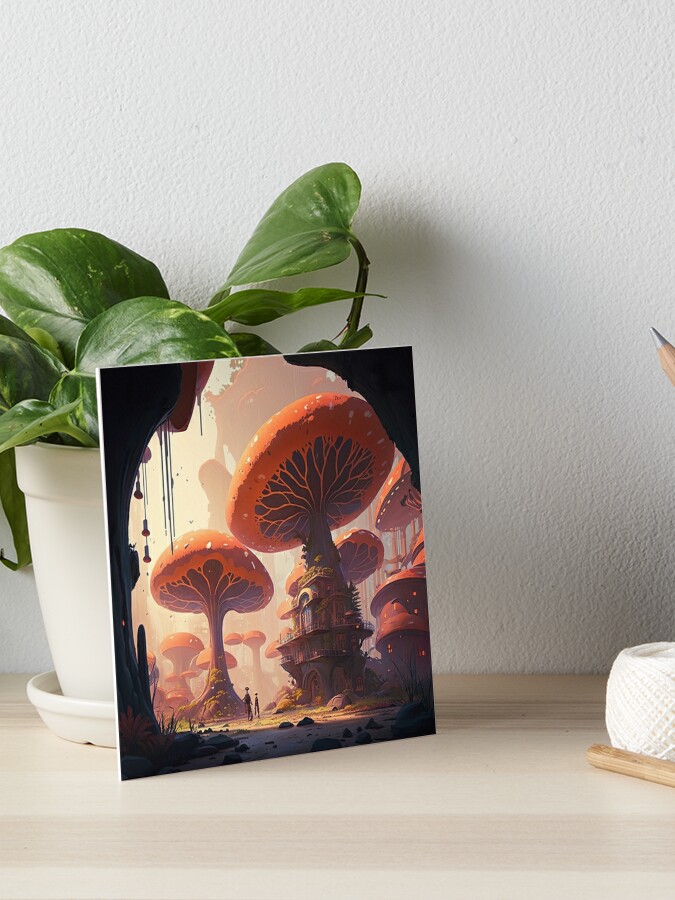The product photograph showcases a small canvas print leaning against a white pot that houses a green leafy plant, set on a flat, light brown wood surface streaked with lighter hues. The background features a solid white wall with a pit-marked texture. The digital print on the canvas depicts a vivid scene of large mushrooms, with their caps appearing orange with white dots and their undersides brown with orange wavy lines, resembling a fantastical village of mushroom houses with treehouse elements. To the right of the canvas, a spool of white string sits next to a brown-handled object, with the tip of a pencil peeking into the frame. The scene is meticulously staged, creating a harmonious and inviting setting that highlights the artistic allure of the canvas print.